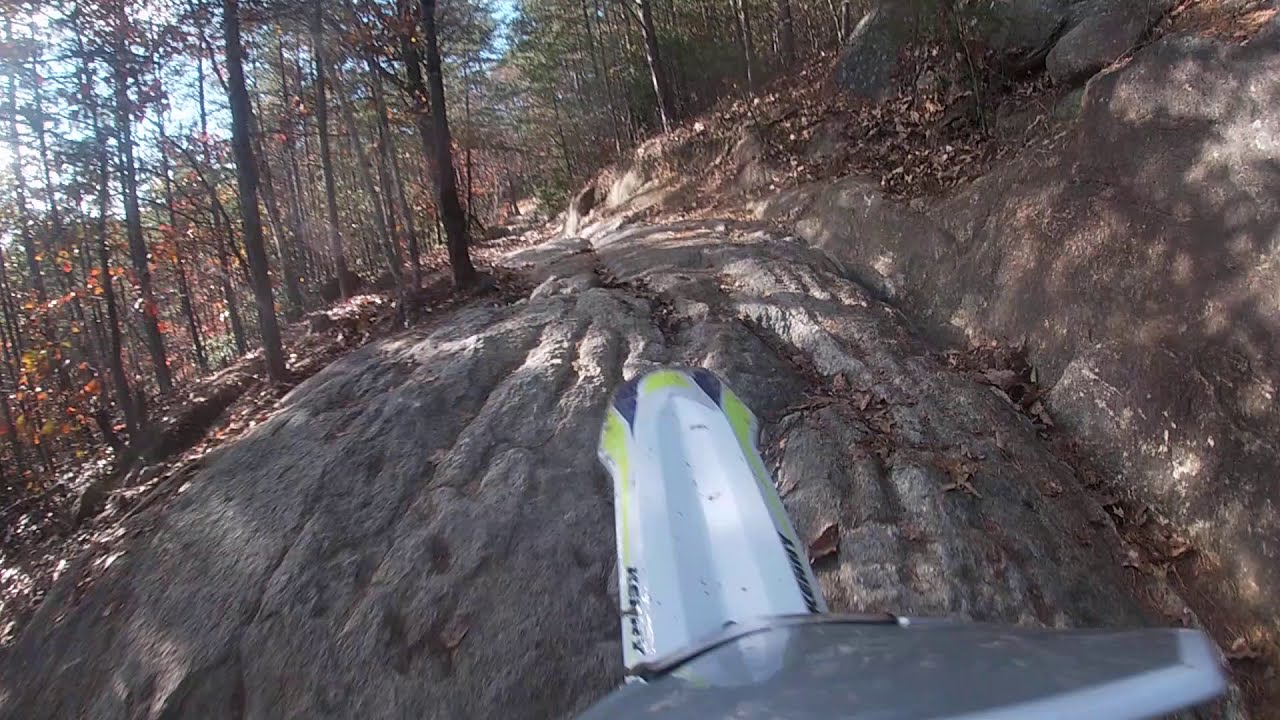The photograph captures a vivid, bright day from the perspective of someone riding a dirt bike along a rugged mountain path. The front fender of the bike, white adorned with green and blue stripes, is clearly visible. The rider navigates over a large, riveted boulder sprinkled with dead leaves and pine needles. The terrain is rocky, with a stone wall rising on the right and a steep cliff sharply descending on the left. Sunlight filters through the sparse, thin branches of trees lining the path ahead, casting intricate shadows. The sky above is a clear blue with white clouds, signaling a crisp fall day. The mixture of green and brown leaves, both fallen and partially clinging to the trees, reinforces the autumn setting.